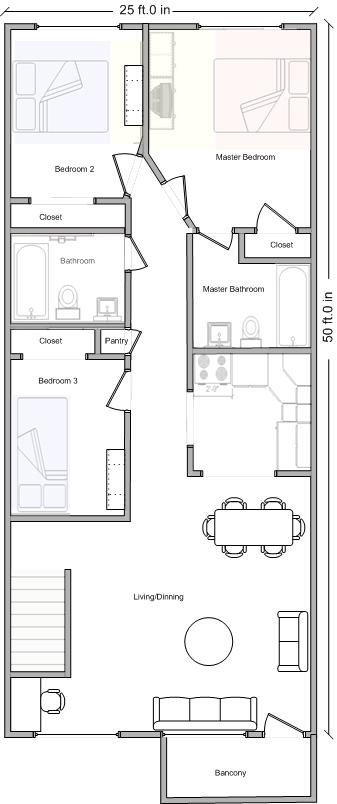Floor Plan of a Residential Area

The floor plan depicts a residential area measuring 25 feet across (east to west) and 50 feet down (north to south). If you orient the top of the plan as north, the layout is as follows:

- **Northwest Side (from north to south)**:
  - A bedroom
  - A closet
  - A bathroom
  - Another closet
  - Another bedroom
  - A staircase

- **East Side (from north to south)**:
  - A master bedroom
  - A closet
  - A master bathroom
  - An unlabeled area presumed to be the kitchen
  - A living and dining area with sketches of a couch, a coffee table, and a dining room table

- In the **southeast corner**, there is a balcony.

Additionally, there is a pantry located off the hallway that connects the east and west rooms. All rooms are distinctly labeled except for the presumed kitchen area.